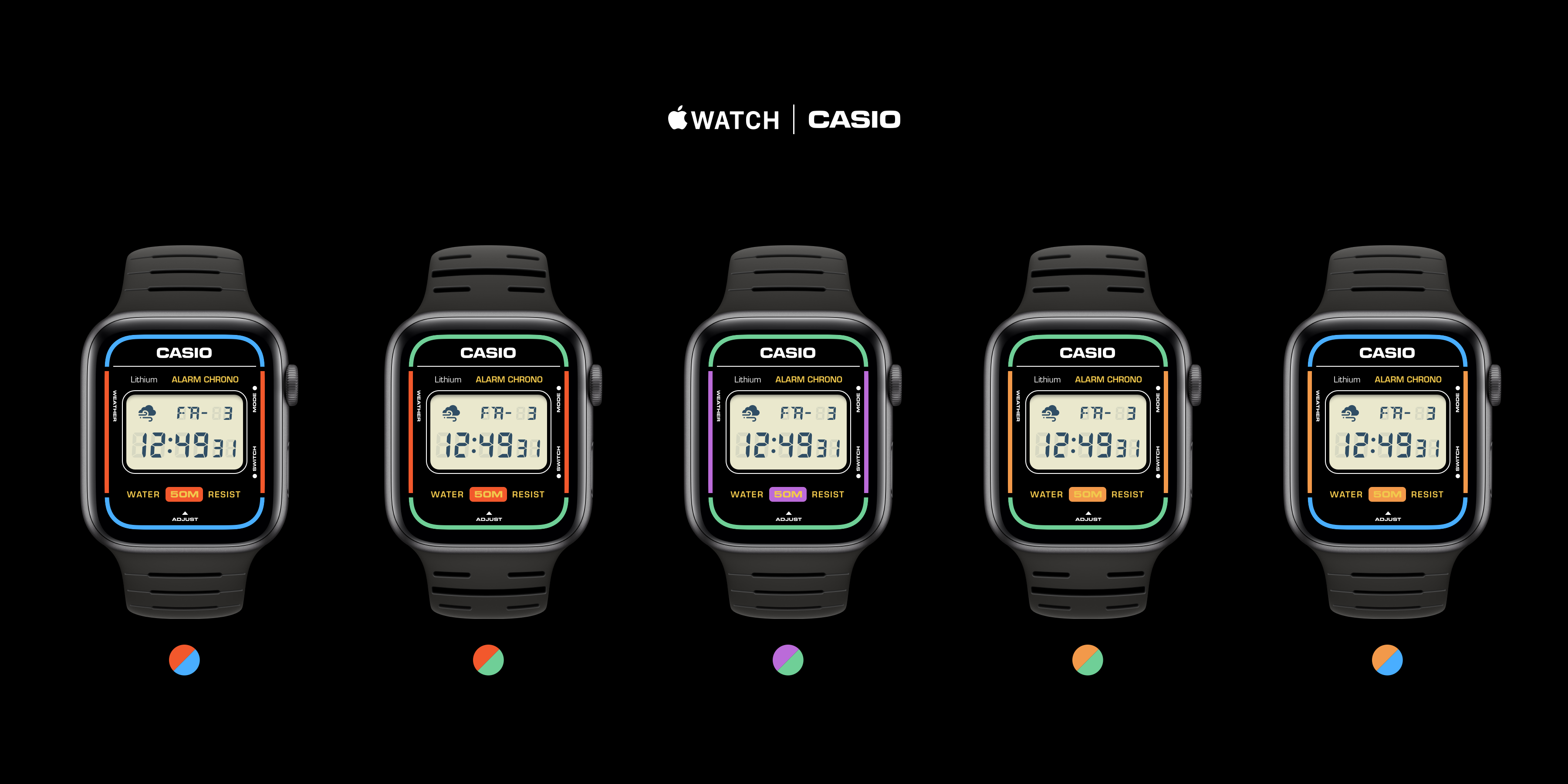The image portrays a sleek advertisement for a collaboration between Apple and Casio, showcasing five distinct Apple Watches, each adorned with black bands and a stainless steel face. All five watches are displayed in a straight horizontal line on a black background, with the branding "Apple Watch Casio" prominent at the top. Each watch features the time "12:49:31" on its screen along with the Casio logo. While the watch bands are uniformly black, the key differentiating feature lies in the colorful borders around each watch face. These borders are in pairs of two colors: the first watch features blue and red, the second green and red, the third purple and green, the fourth orange and green, and the fifth orange and blue. Below each watch, there is a small circle split into the respective two colors, further highlighting the color options available. This image emphasizes the unique customization options available for the watch face borders, catering to consumers looking for personalization in their wearable technology.